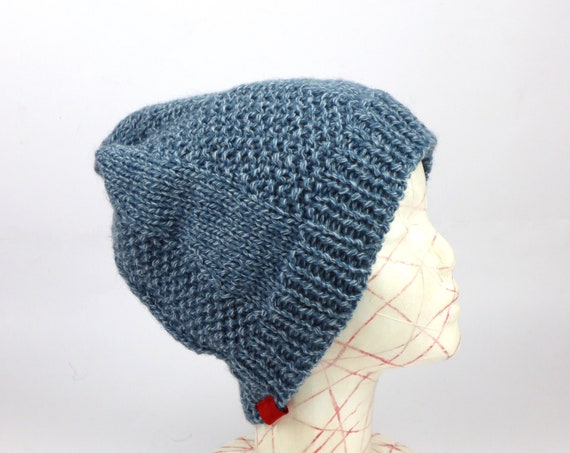This photograph features a close-up of a white mannequin head, displayed from the neck up and facing toward the right. The mannequin is marked with numerous red crisscrossing lines across its face and neck, which create a striking visual effect. It is adorned with a blue knit cap that has a small red tag at the lower edge. The background of the image is a light grayish-white color, providing a neutral setting that contrasts with the mannequin's accents and the colorful cap.